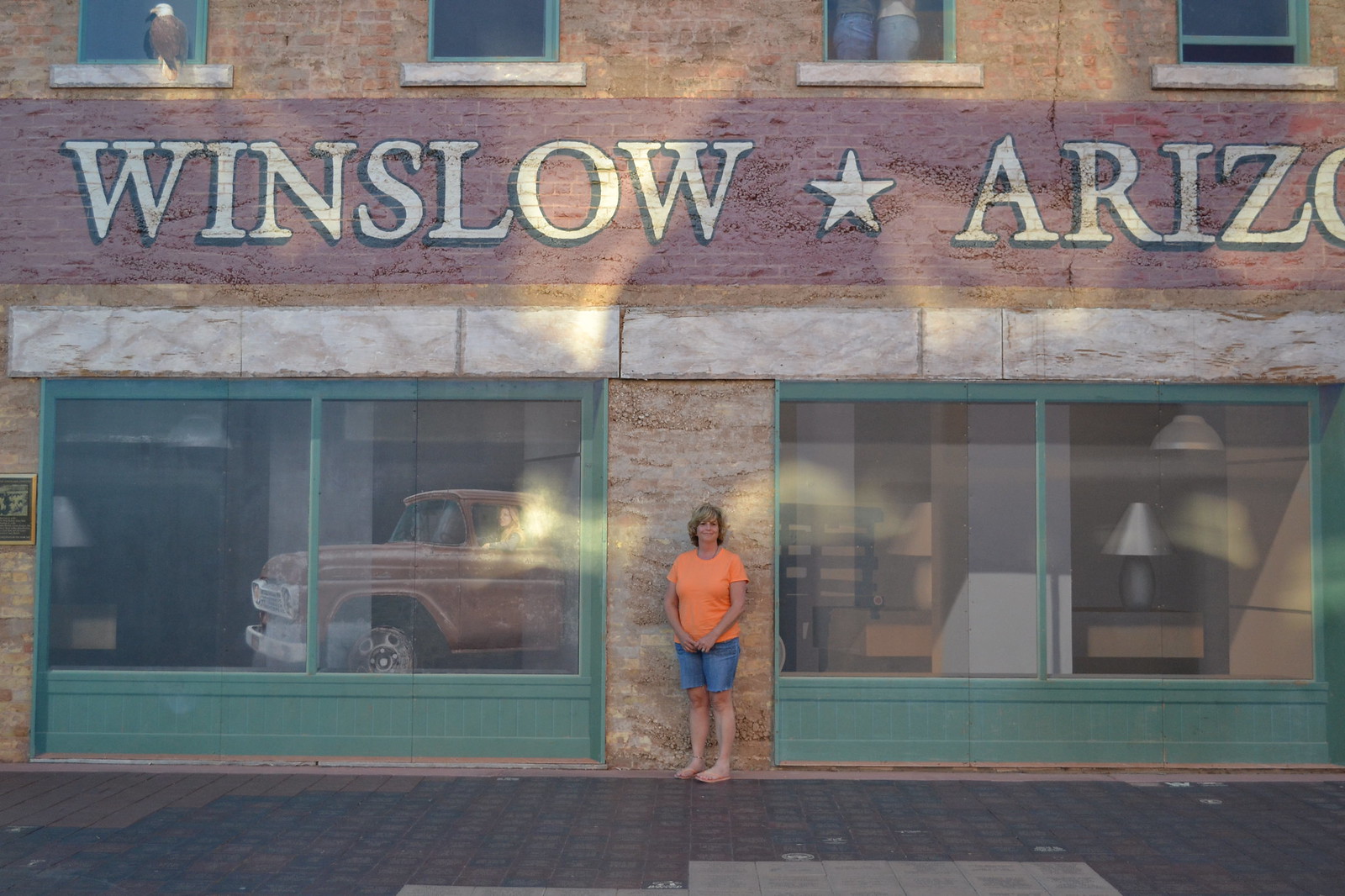In this detailed photograph, a woman is standing outdoors in front of a two-story building with a distinct stone facade. She is wearing an orange short-sleeve t-shirt and denim blue shorts that appear to be cut just above the knee, paired with light peach-colored sandals. Her light brown hair, which has a slight blonde tint, is parted slightly to the left and delicately falls over her forehead. She stands with her hands held together in front of her stomach.

The building behind her features a panel with a stone-like appearance, flanked by large green-framed windows on either side. Above her is a mural that prominently displays "Winslow" in white text, followed by a white star, and then the partially obscured word "Arizona." The mural also incorporates elements reminiscent of a 1950s pickup truck. The upper part of the building shows four brick-framed windows, each with a green frame and a gray bar at the bottom, with the upper right window slightly ajar. A red bar extends across the top section of the brickwork, above which is a brown bar, topped with a red painted strip.

The ground in front of the woman is a mix of light brown and light gray concrete patches, contributing to the textured look of the setting. The foreground features a black sidewalk, creating a stark contrast with the stone and concrete elements around it.